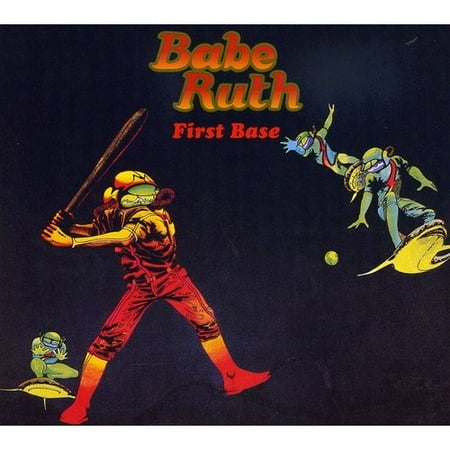The image is a poster set against a solid black background with a title at the top that reads "Babe Ruth" in a retro, bubbly font where the letters gradient from red at the top to yellow at the bottom. Below it, in smaller red letters, it says "First Base."

In the lower left of the image stands a large human figure, ambiguously gendered, dressed in a red suit with red boots and complete scuba diver gear that covers the entire face, ready to swing a large brown bat. Near their foot is a smaller green alien-like figure wearing scuba gear that resembles glasses more than a helmet, floating on a yellow scuba diving board with hands outstretched.

On the right side of the image, two more green alien-like figures are present. These aliens are also wearing blue and green suits with a red stripe, with one standing on a yellow flying saucer and the other hovering above it with outstretched arms, seemingly pitching or preparing to confront the figure with the bat. Beside them lies a yellow ball, indicating they are engaging in a game of baseball while floating on their saucers. 

The text and imagery collectively evoke a surreal scene combining elements of baseball, space, and underwater themes with a touch of the fantastical.